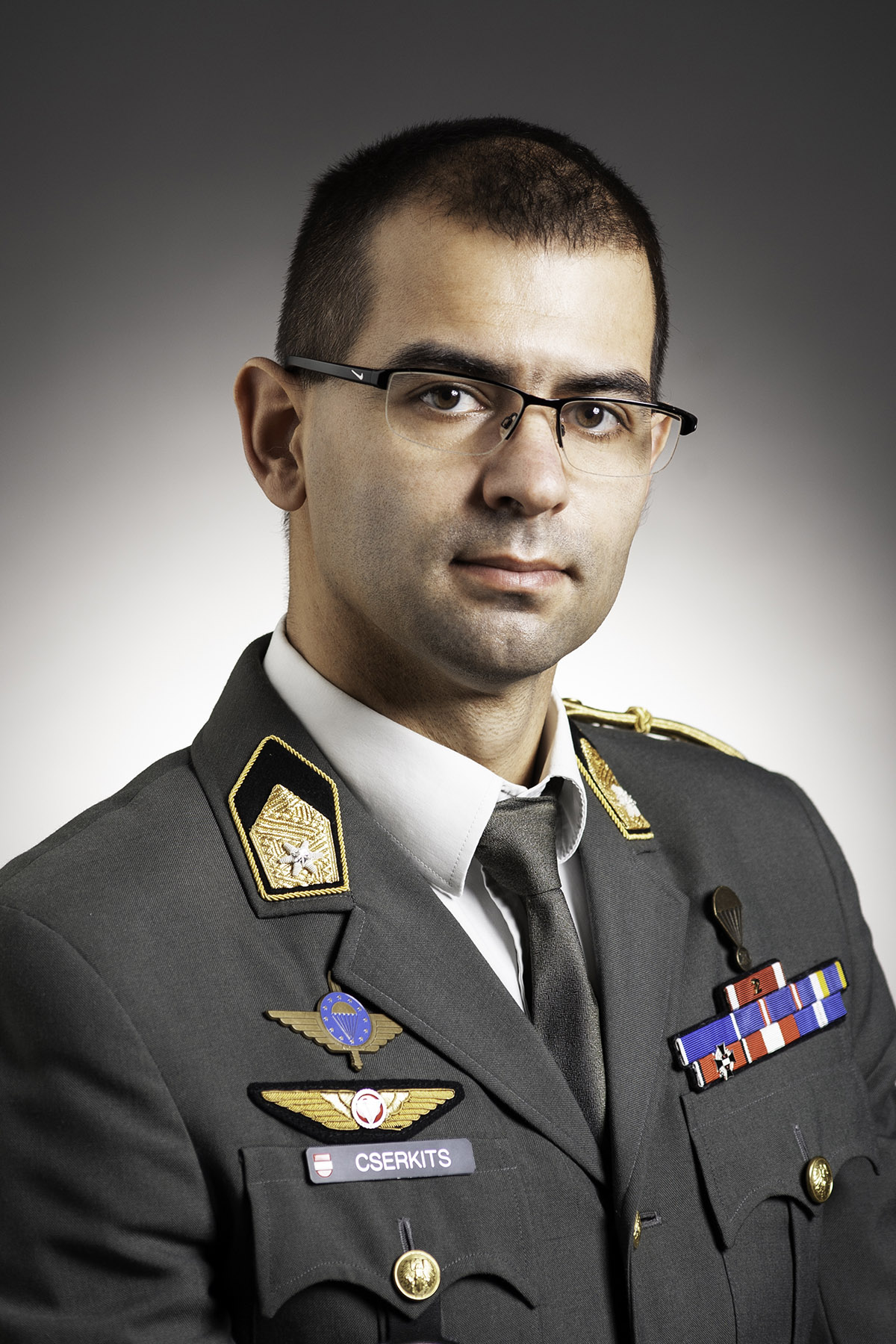The photo features a military man dressed in a distinctive dark grey uniform adorned with various medals and insignia. The man has a smooth, tan complexion and wears glasses. His hair is very short and thin. On his left chest area, multiple medals can be seen, signifying his earned honors. His collar is decorated with rank patches and additional insignias. The right chest area also features an array of medals. Despite the detailed uniform, the specific military branch or nationality remains unclear, as the attire and awards do not appear to resemble American military dress.